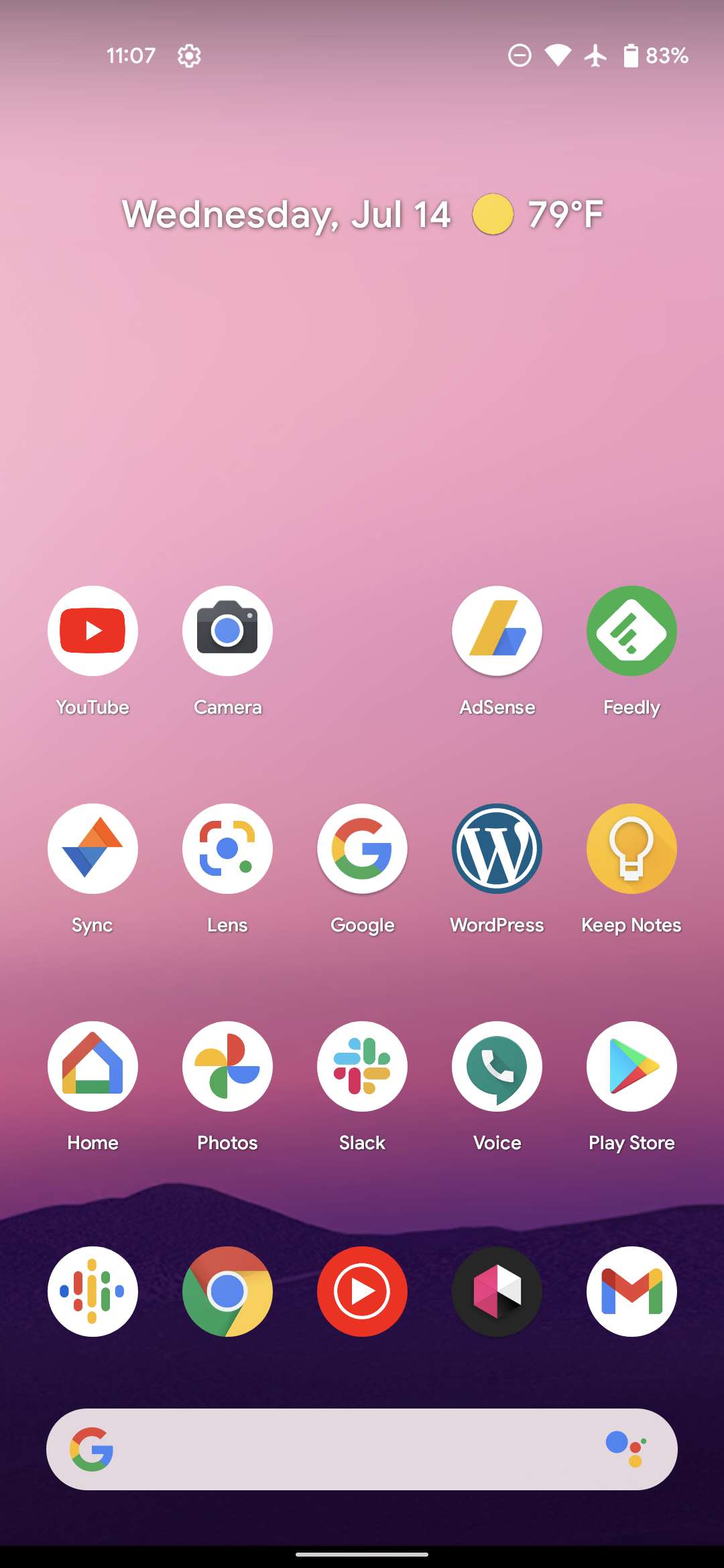The screenshot portrays a mobile phone menu set against a picturesque background gradient, transitioning from a serene pink sunset to a deep purple over the silhouette of black mountains. At the top, the status bar displays the date and weather information: "Wednesday, July 14th, 79°F, sunny."

The screen is organized into a grid with several rows of app icons:

- **Top Row**: YouTube, Camera, AdSense, Feedly.
- **Second Row**: Sync, Lens, Google, WordPress, Keep Notes.
- **Third Row**: Home, Photos, Slack, Voice, Play Store.
- **Fourth Row**: An unlabeled app with rainbow lines in a diamond shape, Google Chrome, an app with a red circle and a white play button, a black logo with hot pink and white diamonds arranged in a hexagonal shape, and Gmail.

These app icons are slightly above the halfway point of the screen. The bottom of the screen houses a prominent Google search bar, complete with the Google "G" symbol on the left and the Google AI symbol on the right. 

This detailed layout captures both the aesthetic appeal and functional arrangement of the phone's menu, making it easy to visualize the screen's organization and the enchanting background setting.